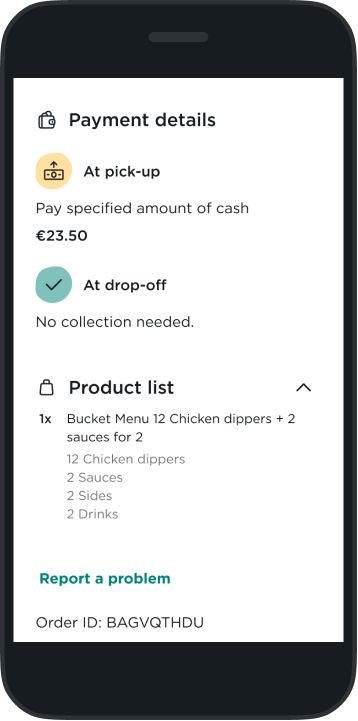A digital receipt is displayed within a phone screenshot, showcasing payment and order details for a pickup item. The receipt header features a wallet icon adjacent to "Payment Details." Below, a yellow circle on the left contains a cash drawing with an upward arrow. To its right, the bold text reads "At Pickup," indicating a cash payment of 23.50 in an unspecified currency upon pickup.

Moving down, a green check mark and a red circle appear on the left side, beside bolded text that states "At Drop Off." Below this, it's noted, "No collection needed." Further down, an icon of a shopping bag appears on the left, adjacent to "Product List."

The detailed order includes:
- 1 Bucket Menu
  - 12 chicken dippers
  - 2 sauces for 2
  - 2 sides
  - 2 drinks

A teal "Report a Problem" link is present near the bottom. The order ID "B-A-G-V-Q-T-H-D-U" is listed at the very end of the receipt. The entire receipt is shown as if displayed on a phone screen, embedded within an image of a phone, suggesting a digital receipt for a chicken dippers bucket menu pickup order.